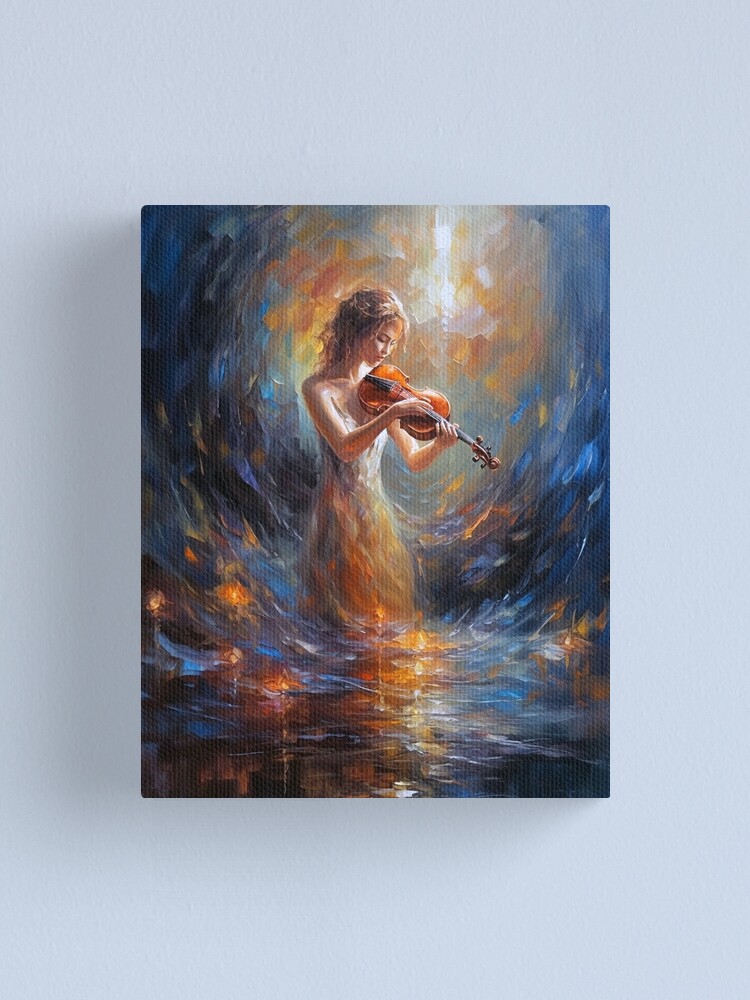This is an abstract oil painting of a young, fair-skinned woman with light red hair, carefully holding and stroking the strings of a medium brown violin. The violin is positioned under her chin while her left hand holds its neck. The painting captures her from a half-profile view, facing right, set against a swirling, vibrant backdrop of oranges, blues, reds, and touches of white. Her depiction and the surrounding colors seamlessly blend together, giving the impression that she is standing in a body of water, with subtle reflections enhancing this effect. The entire image exudes a harmonious blend of colors that bring the piece to life, set on a canvas displayed against a light bluish gray wall. The rectangular painting is devoid of any visible text, animals, or additional people, emphasizing the solitary and serene focus on the young woman and her violin.